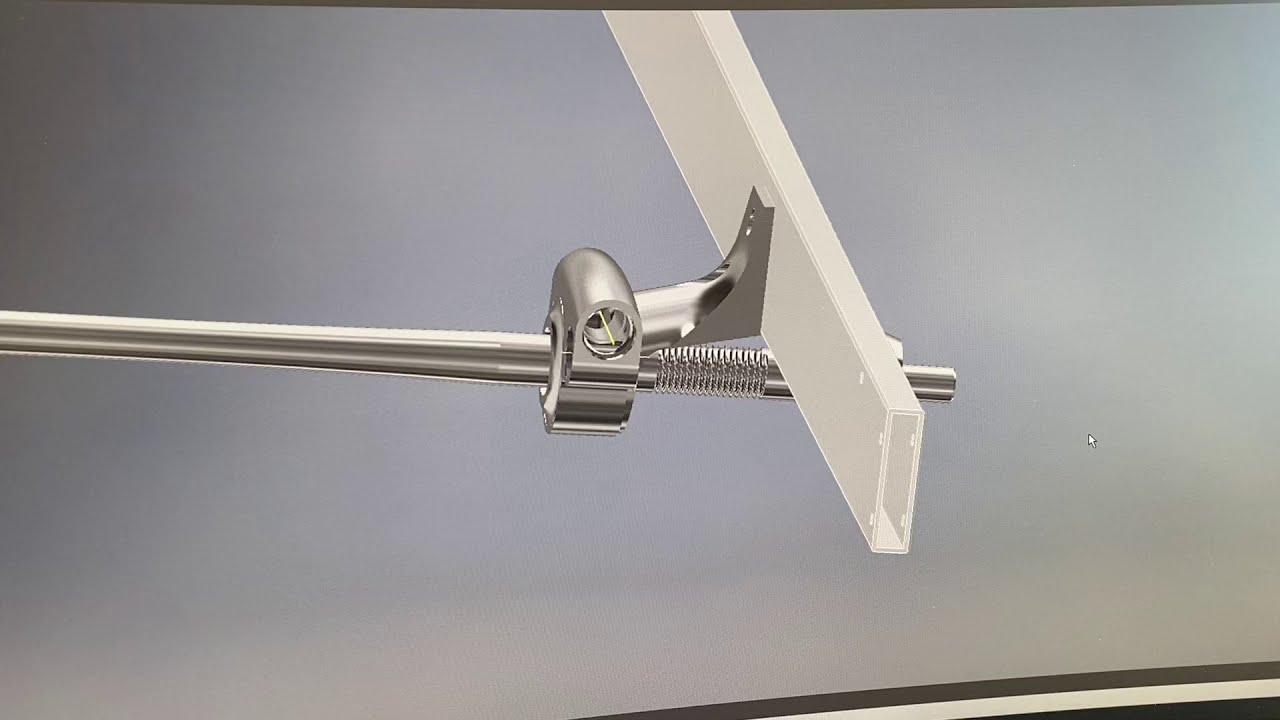This horizontal rectangular photograph captures a bright chrome metal clamp holding a piece of painted white molding, likely made of wood. The clamp, which features a threaded mechanism, is tightly screwed to secure the molding. The bottom of the wood piece is unpainted, revealing its natural texture. The background gradients from darker gray on the left to lighter gray on the right. At the bottom of the image, there is a white stripe flanked by dark lines, possibly indicating the edge of a table with a gray surface. The clamp, emerging from the middle of the frame, and the molding it holds dominate the composition, with no clear indication of the environment beyond these elements.